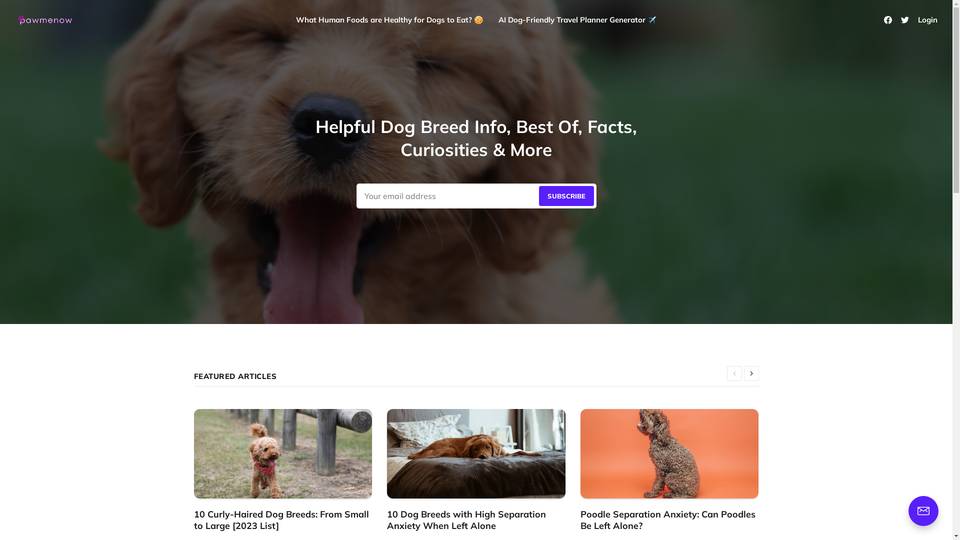**Emergency Information Hub for Dog Owners:**

Explore our comprehensive guide on healthy human foods that dogs can safely eat. Check out the AI-powered dog-friendly travel planner and find essential tips for traveling with your furry friend. Access detailed breed information, fun facts, curiosities, and more. Subscribe to our newsletter with your email address to stay updated on the latest articles and trends.

Featured Articles:
- "10 Curly-Haired Dog Breeds: From Small to Large (2023 List)"
- "10 Dog Breeds with High Separation Anxiety When Left Alone"
- "Managing Low Separation Anxiety: Can Poodles Be Left Alone?"

The webpage is visually appealing with a colorful palette of blue, green, orange, gray, and white. You'll find various images of dogs, beds, and pillows in these colors, creating a vibrant and inviting environment.

(Note: Emphasize the blue, green, white, orange, and gray colors, repeated throughout the page, ensuring a cohesive and visually pleasing design.)